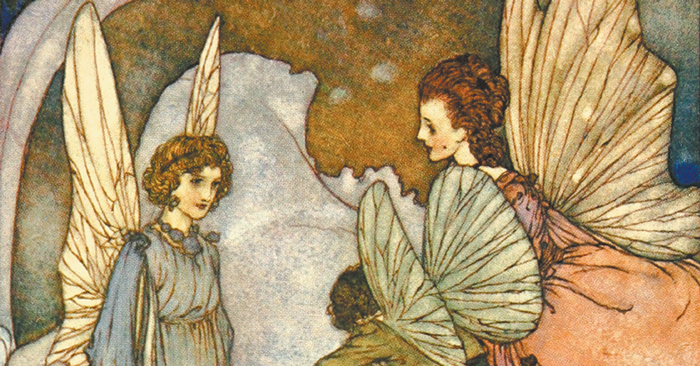This horizontally rectangular painting, rendered in a colorful and artistic style, depicts three winged figures, likely fairies or possibly angels, set against an abstract background featuring gray and brown tones with an arched motif. The scene is a close-up view, focusing on the intricate details of the characters.

On the left, there's a young woman with light brown, curly hair reaching down to her ears, adorned with a black headband. She wears a loose, long-sleeved blue dress and a blue necklace. Her beige fairy wings extend gracefully behind her as she gazes slightly downward.

In the middle, there's another winged figure, possibly a young man or a boy, with brown hair and a green blouse. This individual has smaller, wide light green wings with brown streaks, and their back is partially turned, making their gender indistinct.

On the right, a taller woman with long red hair cascading to her shoulders is clothed in an orange, flowing gown. Her large, light brown wings match the earthy tones of her attire. She is looking towards the woman in blue, adding a sense of connection between the figures.

The artistic piece is painted with a blend of vibrant and earthy colors, emphasizing the ethereal quality of the fairies. There is no text within the image, allowing the visual elements to narrate the scene.